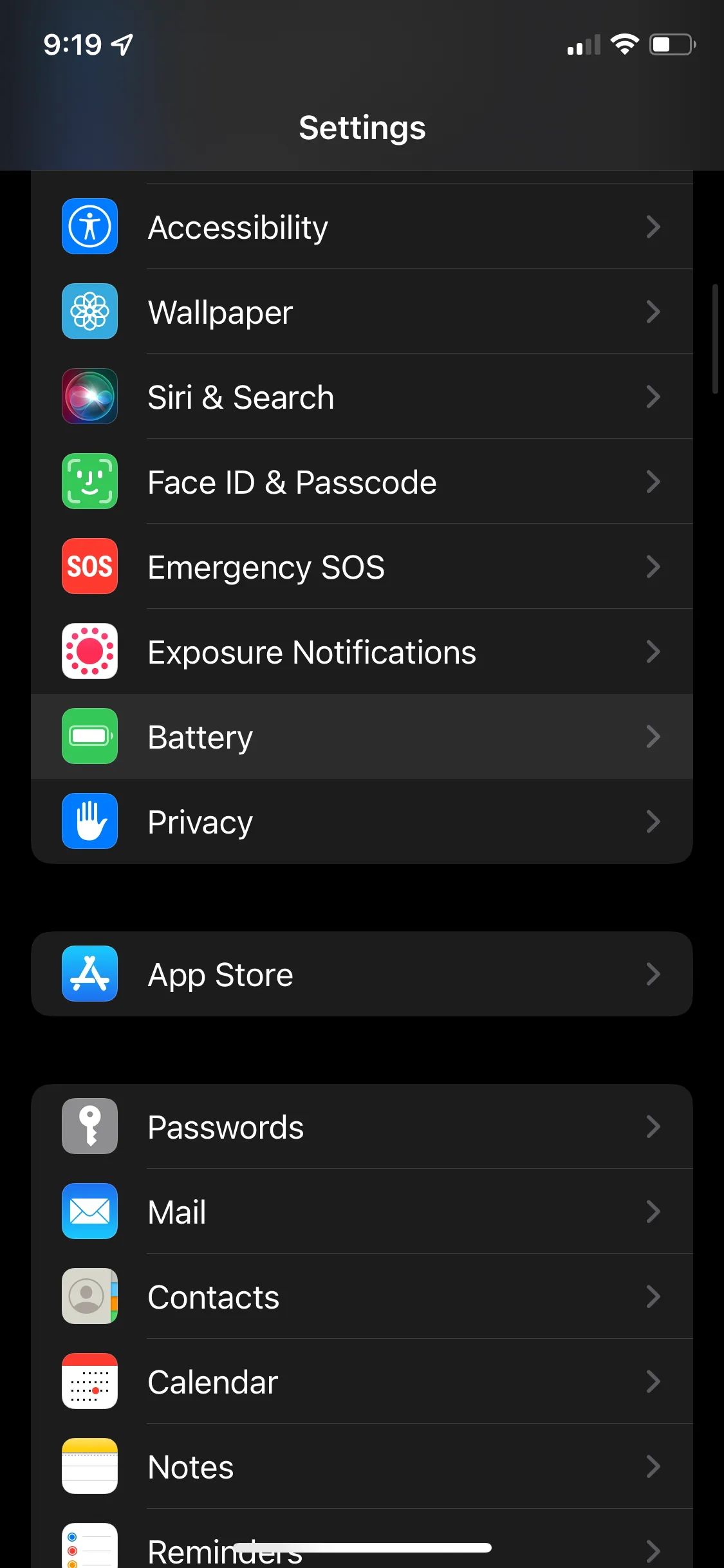The image is a screenshot of the settings page on a mobile phone, specifically an iPhone. The status bar at the top of the screen displays the current time in white font, reading "9:19," along with a small diagonal arrow pointing towards the north-northeast. Positioned to the far right of the status bar are several icons: a signal strength indicator with two bars, a WiFi icon, and a half-full battery icon.

Beneath the status bar, centered near the top of the screen, the word "Settings" is prominently displayed in white font against a black background. This black background persists throughout the settings page, creating a stark, high-contrast interface.

The menu itself features a series of options, each accompanied by an icon on the left side and an arrow on the right, indicating the ability to select and navigate to further sub-menus. The list of menu items, ordered from top to bottom, includes:

1. Accessibility
2. Wallpaper
3. Siri & Search
4. Face ID & Passcode
5. Emergency SOS
6. Exposure Notifications
7. Battery
8. Privacy
9. App Store
10. Passwords
11. Mail
12. Contacts
13. Calendar
14. Notes
15. Reminders

Each menu item is aligned neatly for ease of navigation, enabling quick access to various settings and features of the iPhone.